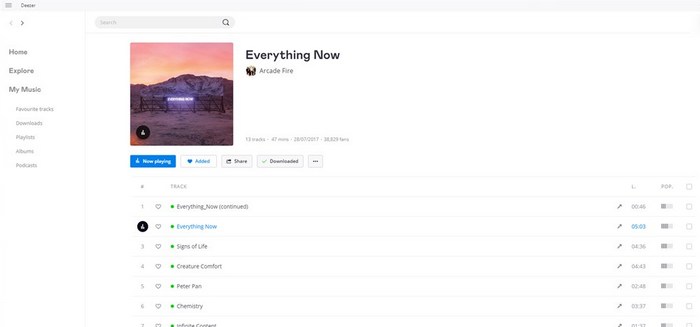This is a detailed screenshot depicting the iTunes desktop application on a completely white background. Dominating the top section is an extensive search bar, with an inconspicuous small word typed in a tiny black font situated towards the far left. Below, on the left side of the interface, runs a vertical panel segregating various categories such as "Home," "Explore," and "My Music," with "My Music" currently selected. Under "My Music," there are five subcategories listed.

On the right side of the panel, a smaller search bar displays the placeholder text "search." Beneath this, a thumbnail represents an Arcade Fire album. Adjacent to this thumbnail, bold black letters spell out "Everything Now," with "Arcade Fire" printed just below it. Further down are four interactive buttons: "Now Playing," which is highlighted in blue, "Added," presented in a white bar with blue text and marked with a heart icon on its left, "Share," and "Downloaded," which is denoted with a green checkmark. Below these buttons, the track listings are organized vertically down the page.